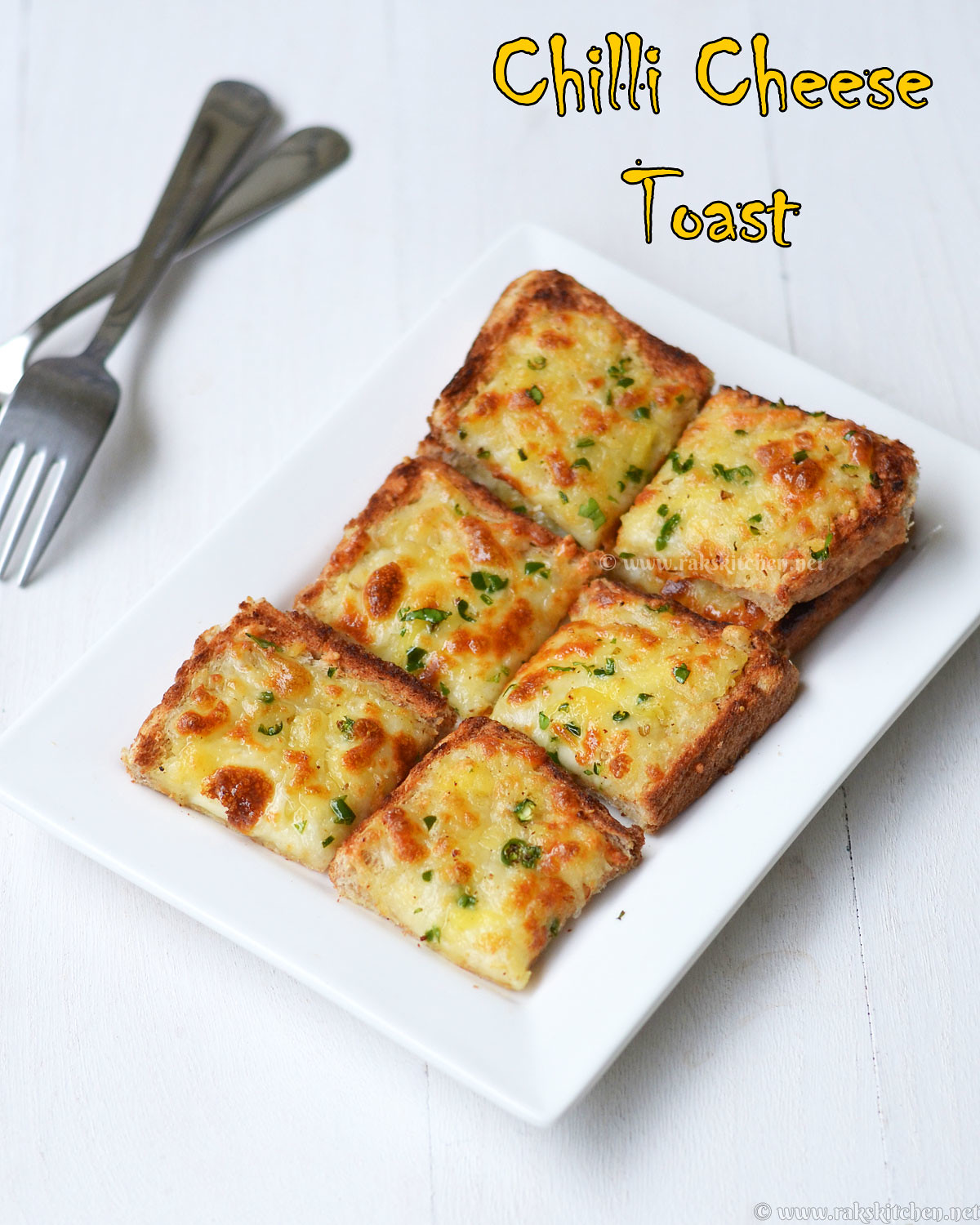This image is a detailed photograph of a dish titled "Chili Cheese Toast," as indicated by the wavy yellow font in the top right corner. The dish comprises six evenly cut pieces of toast arranged neatly on a white rectangular plate. Each square of toast features a topping of melted cheese, which has toasted to a rich golden-brown color, with patches of deeper browns adding texture. The cheese is garnished with green herbs, possibly green onions, adding a touch of color and freshness. The plate is set against a painted white wooden table, with the grain of the wood subtly visible beneath the paint. To the left of the plate, two forks are crossed over each other, ready to be used. In the lower left corner of the image, the website www.raxkitchen.net is noted, lending a professional touch to the presentation.